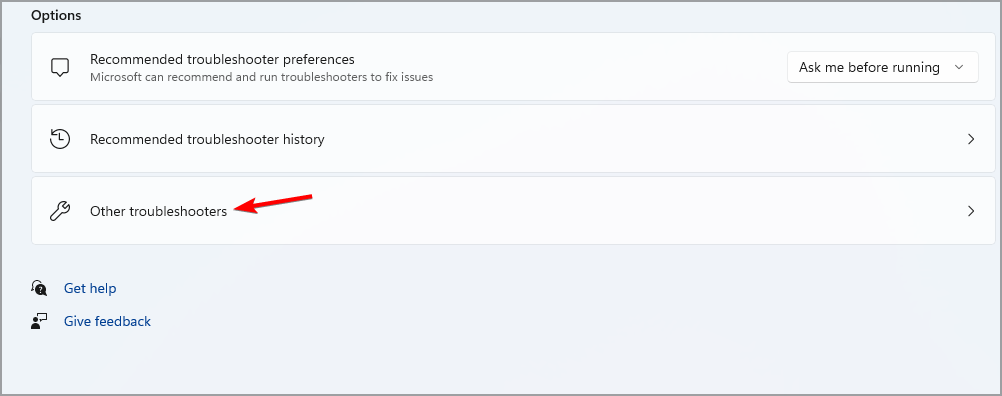The image is a horizontal rectangle with a fine black border surrounding an off-white background. In the upper left corner, the word "Options" is prominently displayed in bold black font. Below this header, there are three crisp white horizontal rectangular sections, each separated by small off-white gaps.

Each section contains an icon to the left and descriptive text in black to the right. The first section features a talking bubble icon accompanied by the text: "Recommended troubleshooter preferences." Underneath this, it reads: "Microsoft can recommend and run troubleshooters to fix issues." To the right of this text is a pull-down menu labeled "Ask me before."

The second section includes a clock icon with an arrow around it, next to the text: "Recommended troubleshooter history." To the right of this is a small "V" icon with the bottom point facing to the right.

The third section has a wrench icon followed by the text: "Other troubleshooters." A bold red arrow points to the "S" in "troubleshooters." All the way to the right of this section is another small "V" icon with its bottom point facing to the right.

At the bottom of the image, against the off-white background, are two phrases in blue font: "Get help" and "Give feedback," each with corresponding icons on the left.